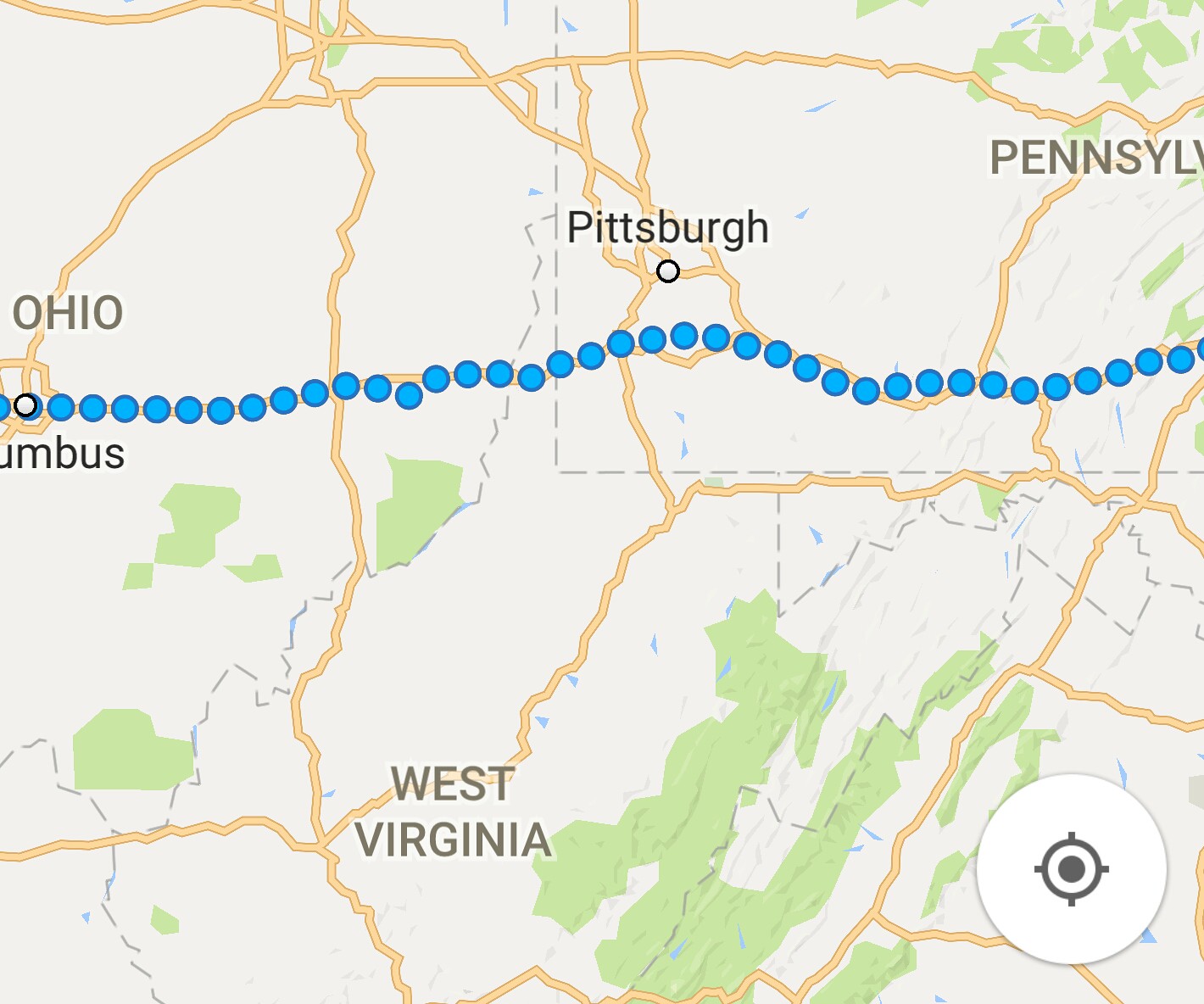This is a screenshot of a map, likely from an older version of Google Maps or Apple Maps, displaying a cream-colored background. The map focuses on the northern region of West Virginia, which is prominently labeled in the middle of the map. To the left, you can see Columbus, Ohio, and towards the top middle, Pittsburgh is marked clearly. On the upper right, the truncated label "PENNSYL" indicates the partial display of Pennsylvania. Running horizontally above West Virginia, a series of blue dots trace a route, presumably along a highway, from Columbus, Ohio, through the southern part of Pittsburgh, and continuing eastward. The roads are highlighted in a light yellow or orange color, while green areas represent forests and landmasses. At the bottom right corner of the map, there's a gray circle with an inner circle and crosshairs, likely serving as a compass or locator symbol. The map indicates travel direction from west to east with no additional text or people present in the image.